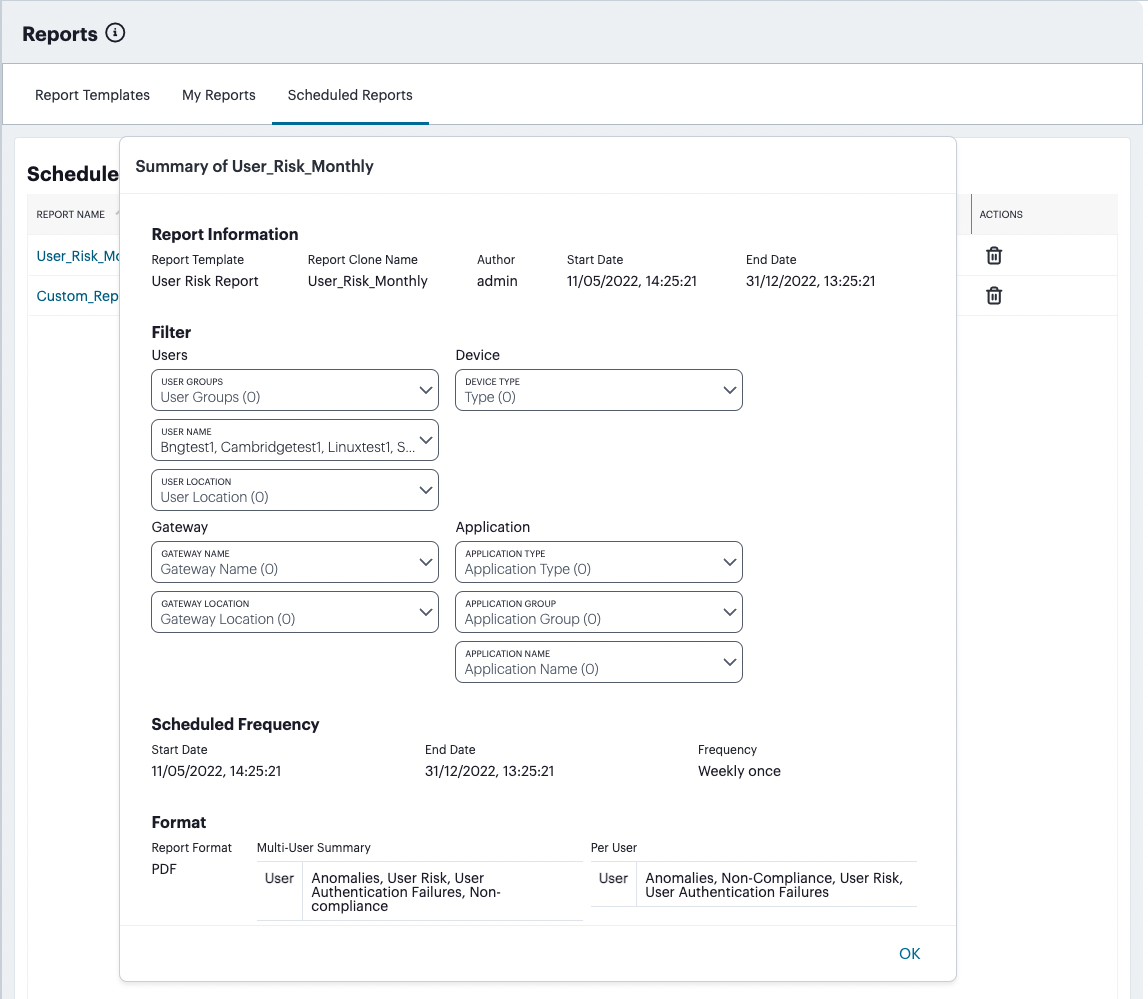The image portrays a screen from an application. At the top, there is a light gray background featuring bold text on the top left that reads "Reports," accompanied by an information icon to the right of this text. Just below, a navigation bar set against a white background includes three categories written in black text. The category on the far right is highlighted, indicated by a small green and blue line beneath the text at the bottom of the background.

Centered on the page is a window titled "Summary of User Risk Monthly" at the top. This section is followed by a header labeled "Report Information." Below this header, various details are displayed. Underneath these details is a list of filters, succeeded by a "Scheduled Frequency" heading, and then a "Format" heading below that.

In the background and slightly behind this central window, another window is visible, marked "Schedule" in the top right corner, featuring a couple of links beneath this heading.